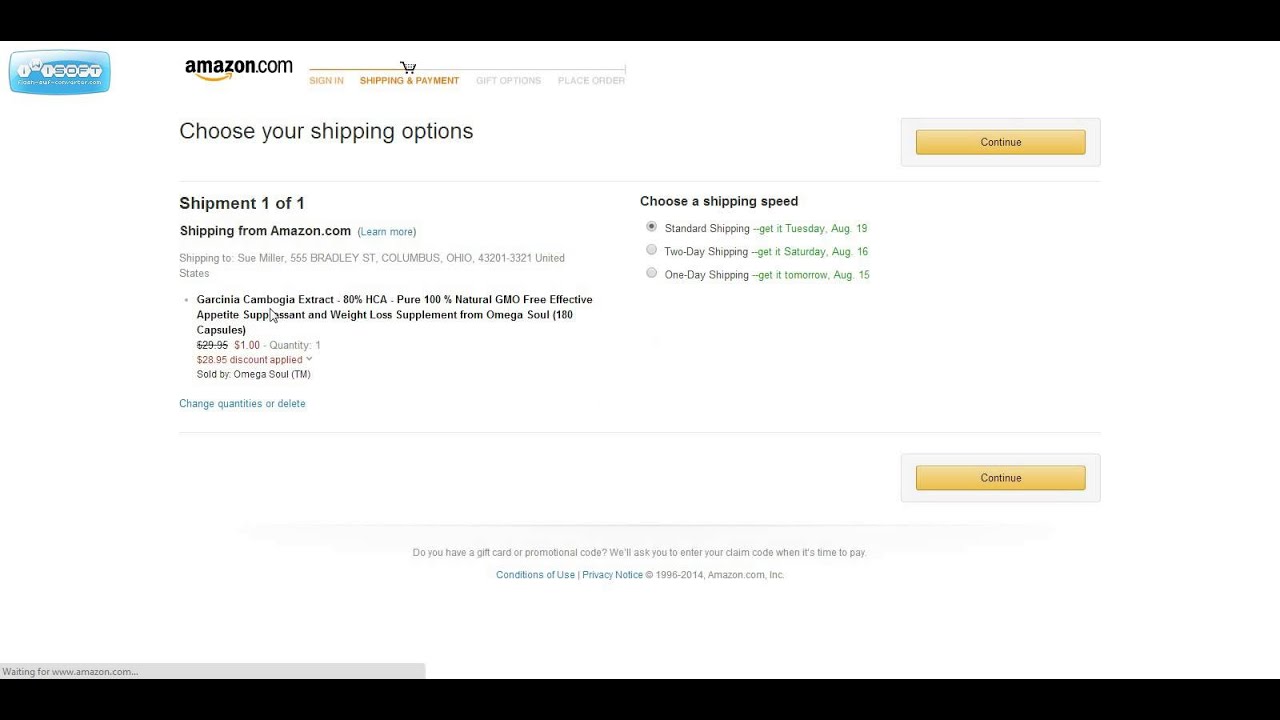This image is a screenshot of an Amazon.com order page, primarily displaying the "Shipping and Payment" section. The layout is wider than it is tall, with black bars running horizontally across the top and bottom of the screen. In the upper-left corner, there's a blue logo with text that is difficult to read. 

To the right of this logo is the prominent Amazon.com logo. Following this are tabs for "Sign In," "Shipping and Payment" (which is currently selected), "Gift Options," and "Place Order," illustrating the sequence of steps for completing a purchase. A shopping cart icon is also visible.

Beneath these tabs, the page instructs the user to choose their shipping options, with a "Continue" button located to the right. The shipment is identified as Shipment 1 of 1, shipping directly from Amazon.com.

The product being ordered is Garcinia Cambogia Extract, an 80% HCA, pure, 100% natural, GMO-free supplement that acts as an appetite suppressant and aids in weight loss. This product is provided by OmegaSoul and includes 180 capsules. The original price of $29.95 is discounted by $28.95, effectively reducing the price to $1. 

The user has selected standard shipping, with an estimated delivery date of Tuesday, August 19th. Alternatives include two-day and one-day shipping options.